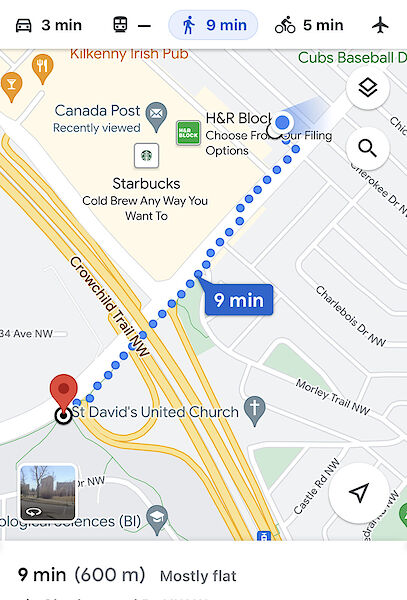This is a cropped screenshot of a Google Maps route overview. The image displays a detailed walking route marked by dots, stretching from the user's current location, represented by a blue circle emitting a blue cone of light at the top right corner, to a red pin indicating the arrival destination. At the top of the screen, travel time options are listed: "3 minutes by car," a dashed line indicating no bus route, "9 minutes by walking" (highlighted, explaining the dotted route), "5 minutes by bike," and a plane icon with no time specified. At the bottom of the map, it specifies "9 minutes, 600 meters, mostly flat." The top right corner of the image features two icons: one for changing the map view and a search icon below it. The bottom right corner contains a reset location icon.